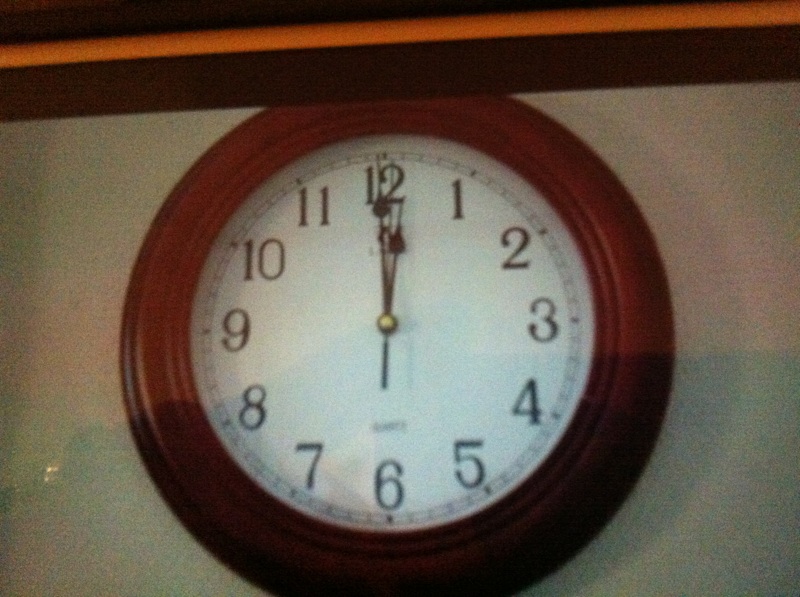This square color photograph showcases a simple, round, walnut-finished wood clock mounted on a gray wall with a distinctive orangey strip and wooden trim at the top. The clock's face is white and uncluttered, displaying Arabic numerals from 1 to 12, with minute increments marked in a concentric circle. The time shown is precisely 12 o'clock, with all three needle-like, thin hands – hour, minute, and the teardrop-shaped second hand – pointing to the number 12. Although the clock’s brand name is positioned above the number six, it remains illegible. The close-up shot captures the overall simplicity and standard design of this analog clock, with its top and bottom edges partially extending out of the frame due to the camera’s proximity.